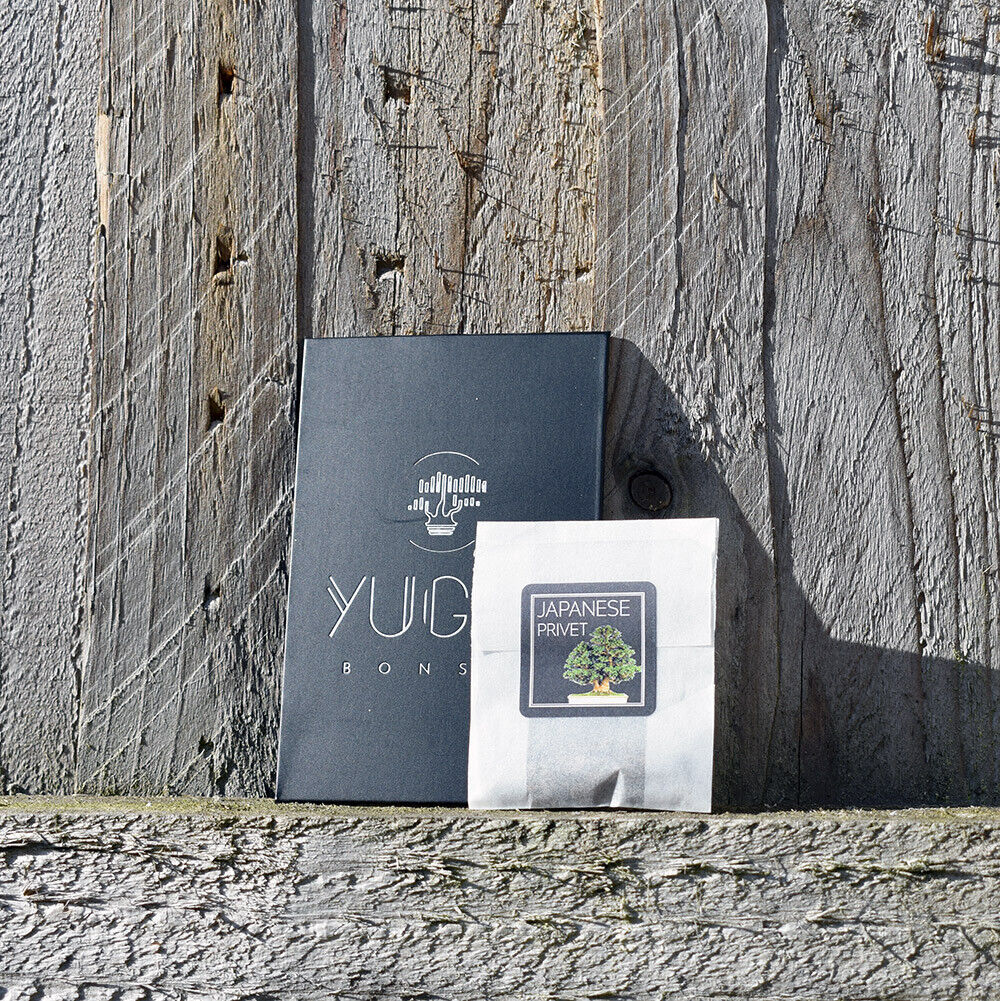This image features a bonsai growing kit presented against an unfinished, weathered wooden background. The setup includes two distinct packages resting on a rough, gray wood surface. The larger package is a flat, black rectangular box adorned with a minimalist line drawing of a bonsai tree in a pot, flanked by two semi-circles. It also includes white text that reads "Y-U-G," with the beginning of "bonsai" visible but partly obscured. The smaller package, identified as a white envelope with a black sticker sealing the flap, is labeled "Japanese Privet" in white text and features an illustration of a small tree with green leaves emerging from a pot. This envelope likely contains materials for growing bonsai, such as seeds or soil. The overall presentation suggests a detailed, well-branded bonsai growing kit designed for enthusiasts.